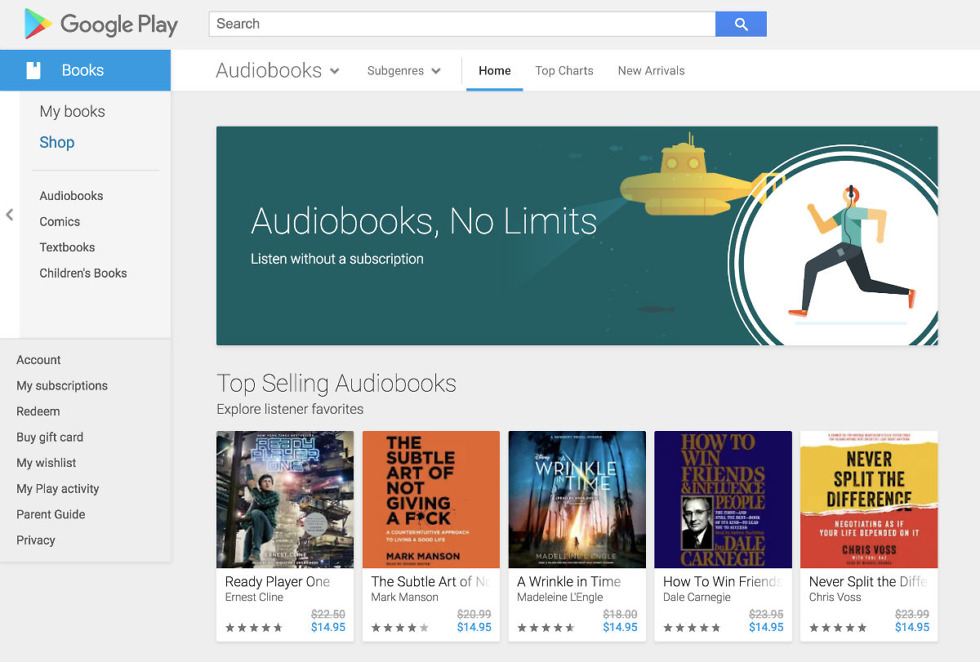This image captures a detailed screenshot of a Google Play webpage dedicated to audiobooks. At the top of the page, various tabs are visible, including Books, Audiobooks, Sub-genres, Home, Top Charts, and New Arrivals. Centrally featured is a prominent banner with the text "Audiobooks, No Limits," and a tagline encouraging users to "listen without a subscription." The banner image depicts a person running with headphones on, along with a submarine casting lights over the words "No Limits," set against a greenish-gray background.

Below this banner, there is a section promoting top-selling audiobooks, inviting users to "Explore listener favorites." Featured titles include "Ready Player One," "The Subtle Art of Not Giving a F*CK," and "A Wrinkle in Time," among others like "How to Win Friends" and "Never Split the Difference."

On the left sidebar, there are navigational links labeled My Books, Shop, Audiobooks, Comics, Textbooks, and Children's Books. Further down, additional options are visible, including Account, My Subscriptions, Redeem, Buy Gift Card, My Wishlist, My Play Activity, Parent Guide, and Privacy.

At the top-left corner of the page, the Google Play logo is prominently displayed, represented by a multi-colored triangle.